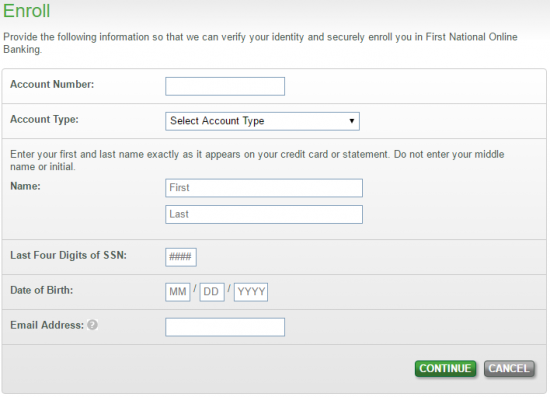The image features a user interface for First National Online Banking enrollment, set against a blue background. At the top, in green text, it reads "Enroll." Below this, a white block contains the instructions: "Provide the following information so that we can verify your identity and securely enroll you in First National Online Banking."

The form below this instruction block is designed with several sections for user input. First, there is a field labeled "Account Number" accompanied by an input box. Next is the "Account Type" section, featuring a drop-down menu prompting users to "Select account type."

Following this, there are fields for the user's name, with specific instructions to enter the first and last name exactly as it appears on their credit card or statement, and to omit the middle name or initial. Separate input boxes are provided for the first and last names.

The form also requests the last four digits of the user’s Social Security Number, with a designated input box, and the date of birth, divided into input boxes for the month, day, and year.

An email address field is presented next, marked by a gray circle and an adjacent input box. At the bottom of the form are two buttons: a green "Continue" button for submission and a gray "Cancel" button.